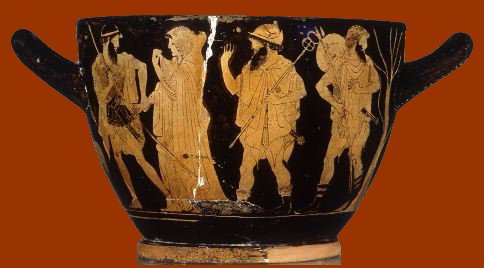This image depicts an ancient piece of Greek pottery, characterized by its deteriorated yet formidable condition. The artifact, resembling a black glazed cup or bowl, bears the marks of age and wear, including a noticeable crack running down its surface. The piece is primarily black, with a tan-colored base and features two small handles protruding on either side. 

The artwork on the pottery is rendered in a yellowish hue, showing four figures: on the far left is a man, distinguished by a beard, holding a pole and clasping the hand of a woman in a long white-yellow dress with a headdress next to him. To their right are two additional men, both equipped with poles, suggesting a scene of exploration or hunting. There is also a tree depicted on the far right side. The background of the image is a medium brownish-orange color, providing a warm contrast to the black and yellow of the pottery, further enhancing its ancient and rustic aesthetic.